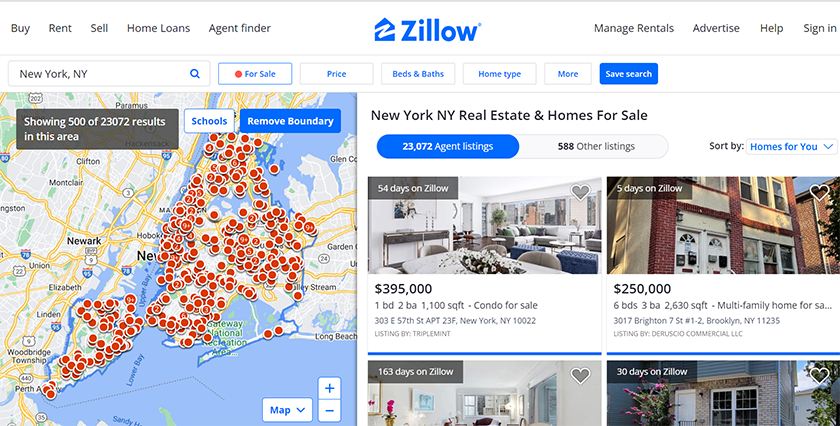This detailed caption for the Zillow website screenshot image captures all key elements effectively:

---

The screenshot displays the Zillow homepage, prominently featuring the Zillow logo at the center—an iconic blue word "Zillow" accompanied by a blue house with a stylized "Z" shape within it. On the top left, there are five navigation categories arranged from left to right: Buy, Rent, Sell, Home Loans, and Agent Finder. On the top right, there are four more categories: Manage Rentals, Advertise, Help, and Sign In.

Below these categories on the left, there is a search bar with "New York, NY" entered as the location. Adjacent to the search bar is a partial map of New York City, characterized by a dense array of at least 100 red dots indicating property listings. A dark gray rectangle beneath the search bar notes, "Showing 500 of 23,072 results in this area." Right next to this information are options to view schools and to remove the search boundary.

To the right, the page highlights "New York, NY Real Estate and Homes for Sale," with a total of 23,072 agent listings matching the search criteria. The first property listing displayed is priced at $395,000, followed by another listing at $250,000. Each property includes an image, either of the interior or exterior, and the listing dates are visible below these images. The entire interface is set against a clean, white background, making the elements stand out clearly.

---

This comprehensive caption covers the visual and textual details displayed in the Zillow screenshot.